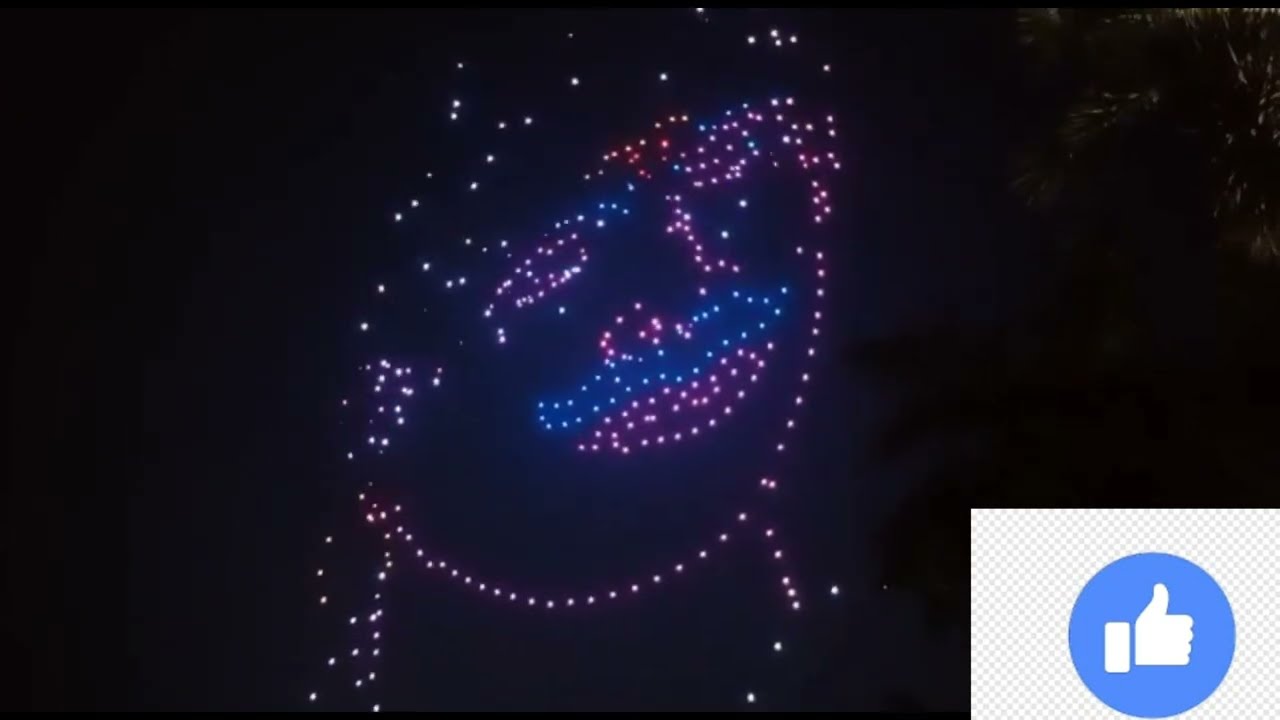In this captivating digital image, a stylized, cartoon-like portrait of a person with a mustache is intricately formed using a dazzling array of lights against a stark black background. The face is composed primarily of varying hues of red, pink, and white lights, with distinct blue lights highlighting the mustache and possibly the eyebrows. The portrait also includes a faint outline of a shirt and what might be a hat above the eyes, further enhancing the human likeness. To the lower right of the image, a prominent thumbs-up icon, reminiscent of the Facebook 'like' symbol, is embedded within a blue circle, accompanied by a subtle mesh pattern of light blue squares. The overall effect is strikingly reminiscent of a constellation or drone light show, where the lights have been meticulously arranged to create a visually stunning, digitally-rendered display.